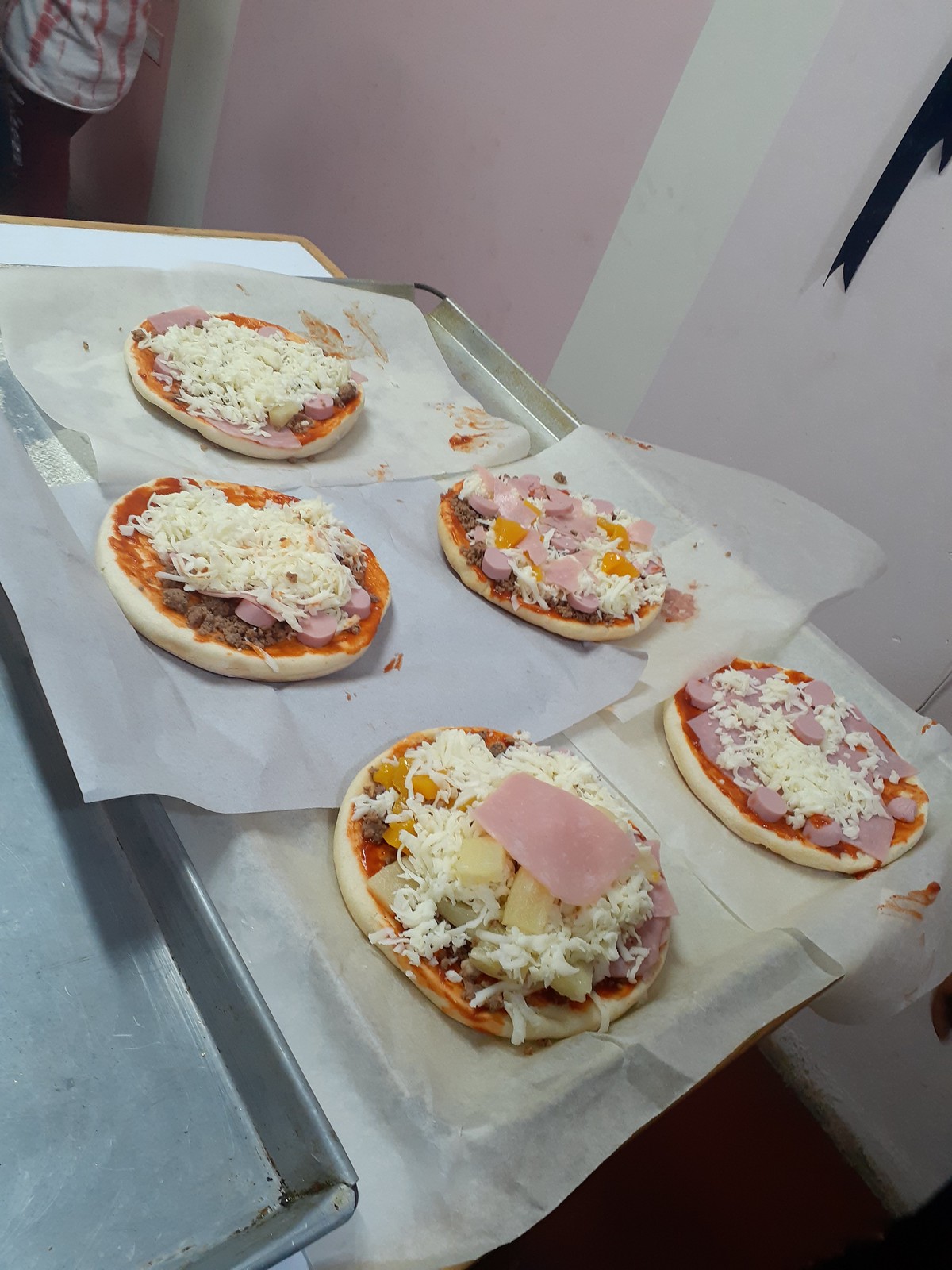The photograph captures five uncooked mini pizzas meticulously arranged on a white parchment paper, which rests upon a silver baking sheet. These small pizzas are diverse in their toppings, featuring generous amounts of shredded cheese, which are notably placed on top of ingredients like ham, chopped and rough-cut peppers, pineapples, and beef. The pizzas are positioned closer to the right side of the tray, forming a neat pattern. Adjacent to this tray is an empty silver tray. The backdrop features a wall with pink, white, and lilac shades, enhancing the scene's colorful and detailed composition.